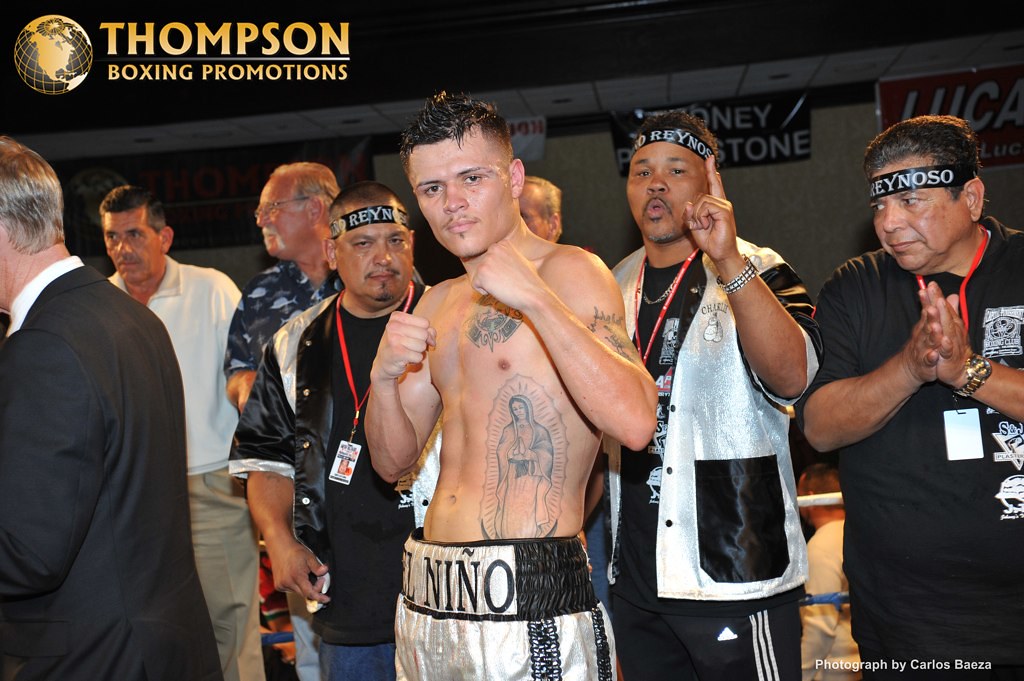In this promotional image for Thompson Boxing Promotions, prominently displayed in gold text at the top left corner alongside a golden globe logo, the central figure is a shirtless boxer with short, spiked hair, a wisp of a mustache, and a soul patch. The waistband of his white shorts, accented with black stripes, features the name "El Nino" in bold black letters. His bare chest showcases multiple tattoos, including a conspicuous depiction of the Virgin Mary on his lower left chest. Striking a fighting stance with his fists raised, he is flanked by a trio of men, likely his trainers or managers, all clad in black and white attire and wearing black headbands inscribed with the word "Reynoso." The man to his immediate left dons a black shirt, black pants, a lanyard around his neck, and a black bandana with white letters over his forehead, his hands clasped in front of him. To his right stands another individual in a black shirt, a white vest, and black shorts, while over the boxer's right shoulder is a third man with a red lanyard, wearing a short-sleeved black and white shirt paired with blue jeans. Additional individuals and incidental people populate the background, which is adorned with various banners and promotional materials. The image is credited at the bottom right corner with the text "Photographed by Carlos Baeza."